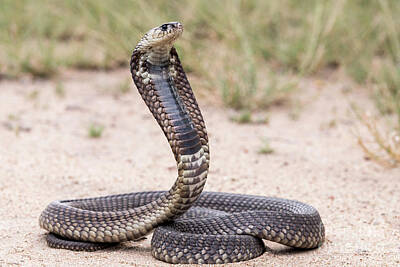The photograph captures a brown-bodied cobra, distinctly recognized by its hooded neck, coiled up and seemingly vigilant. Its beady black eyes are fixed towards the upper right, appearing alert but not aggressive, as its tongue is not extended. The cobra's scales display a unique pattern, with a purplish strip running from its neck down to its belly. The snake is depicted on a sandy, gravelly surface, hinting at a wild, natural habitat rather than a captive environment. Behind the cobra, vibrant green grasses contrast against the earthy tones, further emphasizing the snake's natural setting. The professional quality of the image, with its strong depth of field, suggests it was taken by a skilled nature photographer.